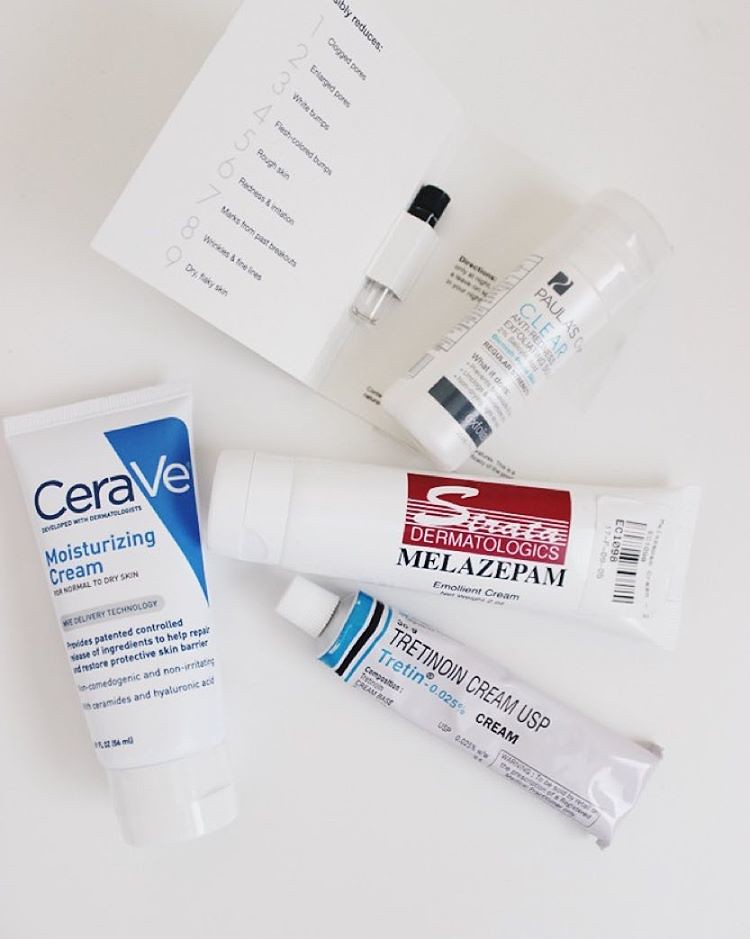"Color photo on a bright white background showcasing an array of dermatologic creams, ointments, and medications under excellent lighting conditions. At the top left, a diagonally placed label, partially visible, likely reads 'Notably Reduces.' The label lists nine benefits, including 'clogged pores,' 'enlarged pores,' and 'rough skin.' The list is attached to a clear vial with a black cap, presumably a product sample. Adjacent is a cylindrical white container with a clear lid from Paula's Choice, a recognizable skincare brand.

Running horizontally across the middle is a white squeeze tube labeled 'Strata Dermatologics' in white text on a red background, identifying it as 'Melazopam Emollient Cream.' The tube features a flip-top cap on the left and a price tag on the right. Below, a foil ointment tube, white with blue and black bands, is labeled 'Tretinoin Cream, USP,' adorned with the trademark symbol and other fine print.

In the bottom left, a white squeeze tube of CeraVe Moisturizing Cream is highlighted. The prominent 'CeraVe' logo sits atop the tube, with the 'V' and 'E' encased in a blue triangle. The description in blue text mentions a patented, controlled ingredient designed to help maintain the skin's protective barrier. This curated collection of skincare essentials aims to target a variety of dermatological concerns."